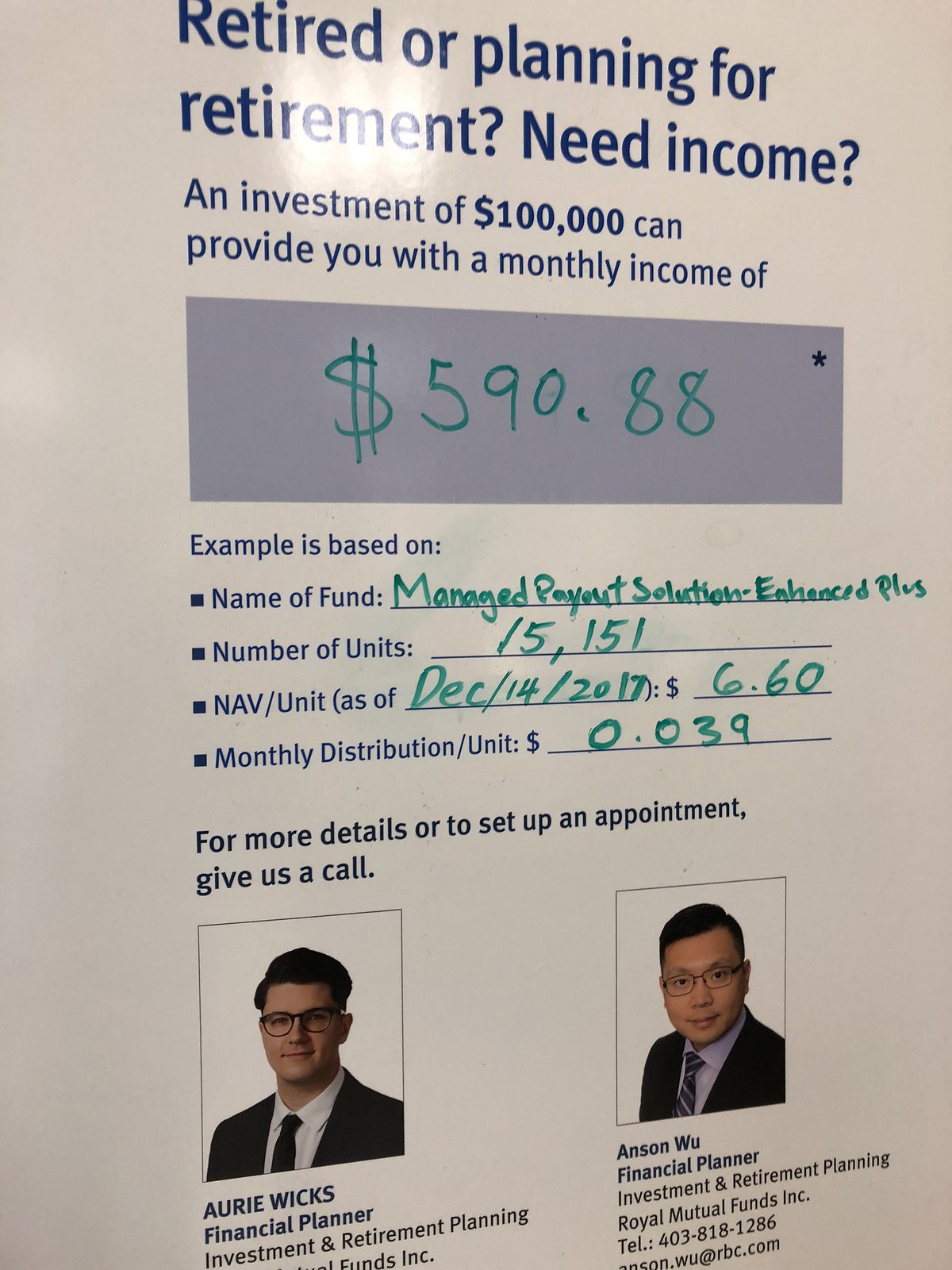This image features a detailed informational poster on investment options for retirement, prominently displaying the headline “Retired or Planning for Retirement? Need Income?” Written in blue text at the top, it explains that an investment of $100,000 can provide a monthly income of $590.88, which is hand-marked in green pen within a gray rectangular box. Below this, further blue text details an example based on a specific fund: "Managed Payout Solution Enhanced Plus," with units listed as 15,151, a NAV per unit of $6.60 as of December 14th, 2017, and a monthly distribution per unit of $0.039. To the side, more information about the example is handwritten in green ink, including the investment name and figures.

The lower section of the poster includes two photographs: one of Ori Wicks, a financial planner, on the left, and Anson Wu, a financial planner specializing in investment and retirement planning for Royal Mutual Funds, Inc., on the right. Ori Wicks is depicted with black hair, glasses, a black suit, and a black tie. Anson Wu, with short black hair, is shown wearing glasses, a black suit, a purple shirt, and a tie. Contact details for Anson Wu, including his telephone number and email address, are provided beneath his photo. The entire composition is set against an off-white background, offering a professional and informative visual aid for those planning their retirement income.